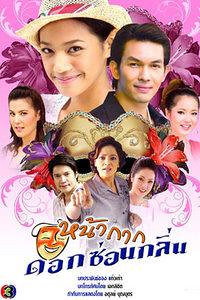This vibrant entertainment flyer, likely promoting an Asian film or performance with possible Thai origins, features a dynamic composition against a pink and purple floral background. Central to the image is a smiling man with short brown hair wearing a blue shirt, situated among a group of individuals. Foregrounded is a woman in a purple shirt pointing, flanked by a man to her left and another woman to her right. Above them, a gold crown rests, highlighting its significance. Inside this crown are additional figures: a girl wearing a hat and a gentleman smiling warmly, with two more females positioned to their left and right. The entire scene is encircled by intricate floral patterns in shades of pink and red, enhancing the visual appeal. At the bottom of the flyer, an orange and yellow mask logo with a cheerful expression stands out, accompanied by bold orange text likely signifying the event's title, and further blue and black script in Thai. Additionally, a logo featuring the number three is positioned towards the lower section. The colors throughout the poster range widely, including pink, white, gray, green, red, purple, and various shades of blue, making the flyer both eye-catching and vividly detailed.